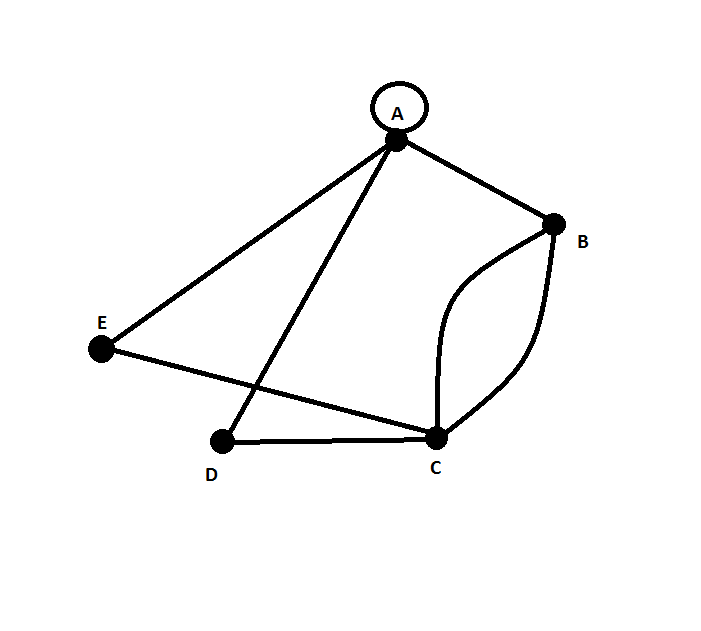This black and white graphic image, reminiscent of illustrations found in a math textbook, features a set of interconnected lines with notable simplicity yet intricate detail. Five primary connection points labeled A, B, C, D, and E are marked by black dots at each intersection of the lines. The image includes both straight and curvy lines, with the straight lines forming the majority. Between points B and C, two curvy lines arc gracefully, resembling the outline of a crescent roll. Despite its non-symmetrical and irregular configuration, the arrangement forms a connection of points that collectively could be considered a polygon. The white background ensures the focus remains on the stark, precise black lines and dots, creating a clean and educational visual.